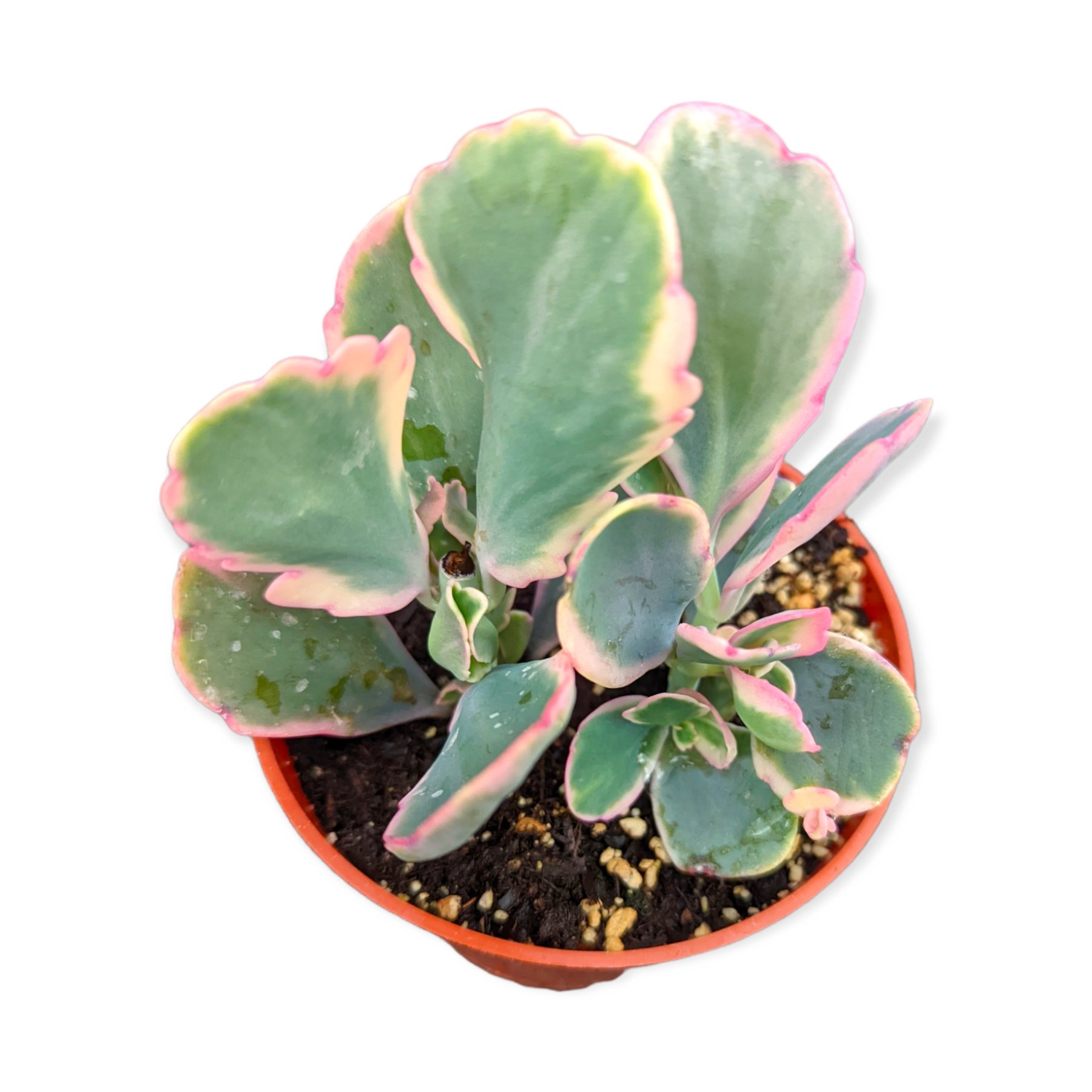This is an aerial, top-down view of a vibrant succulent plant, meticulously captured in a close-up photograph. The plant is nestled in a reddish-orange container, possibly made of plastic, though the exact material isn’t discernible. The container's rim is visible, surrounding the dark potting soil enriched with tiny, white nutrient specks. The succulent’s thick, lettuce-like leaves dominate the image with their green and cream hues, each edge uniquely tinged in delicate pink and interspersed with subtle yellow tones. The background has been completely whited out, emphasizing the contrasting colors and intricate details of the plant and its container.